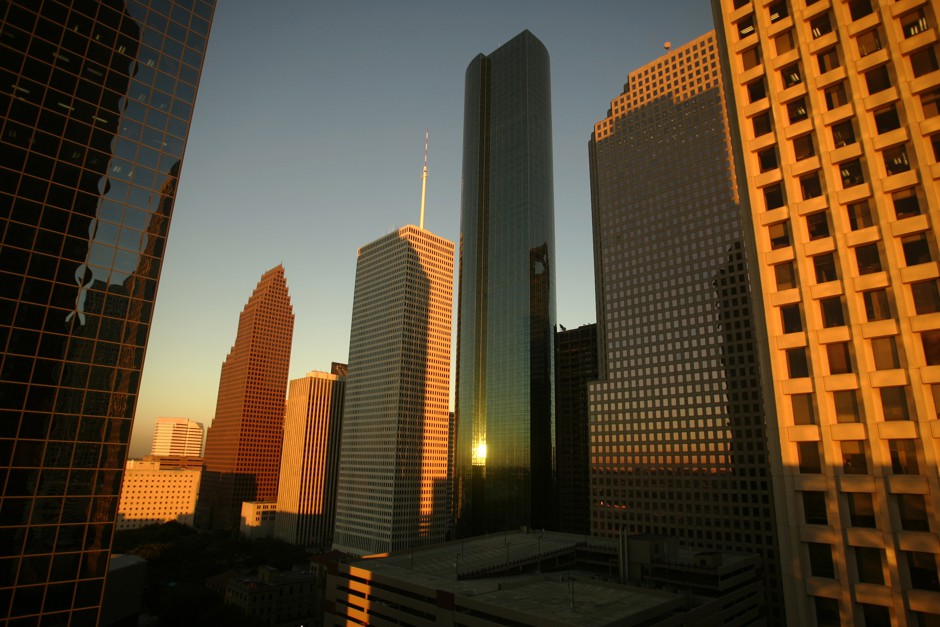The image is a professional color photograph of a city skyline, likely taken from a building window or by a drone during golden hour. The composition stretches more horizontally than vertically, offering a detailed view of several skyscrapers against a clear blue sky. To the right, a concrete skyscraper with at least 17 stories stands adjacent to a modern glass and concrete building. Below these, a lower structure resembling a parking garage is visible. Dominating the center, a tall, glass obelisk-like skyscraper rises high, while another shorter concrete and glass building with a pole on top stands nearby. The left side features a glass skyscraper, its fluorescent office lights visible and giving the illusion of the building leaning inward due to the angle. The overall scene is bathed in the sun's golden light, creating a dramatic contrast between illuminated facades and areas cast in shadow, and the atmosphere appears slightly smoggy closer to the horizon.